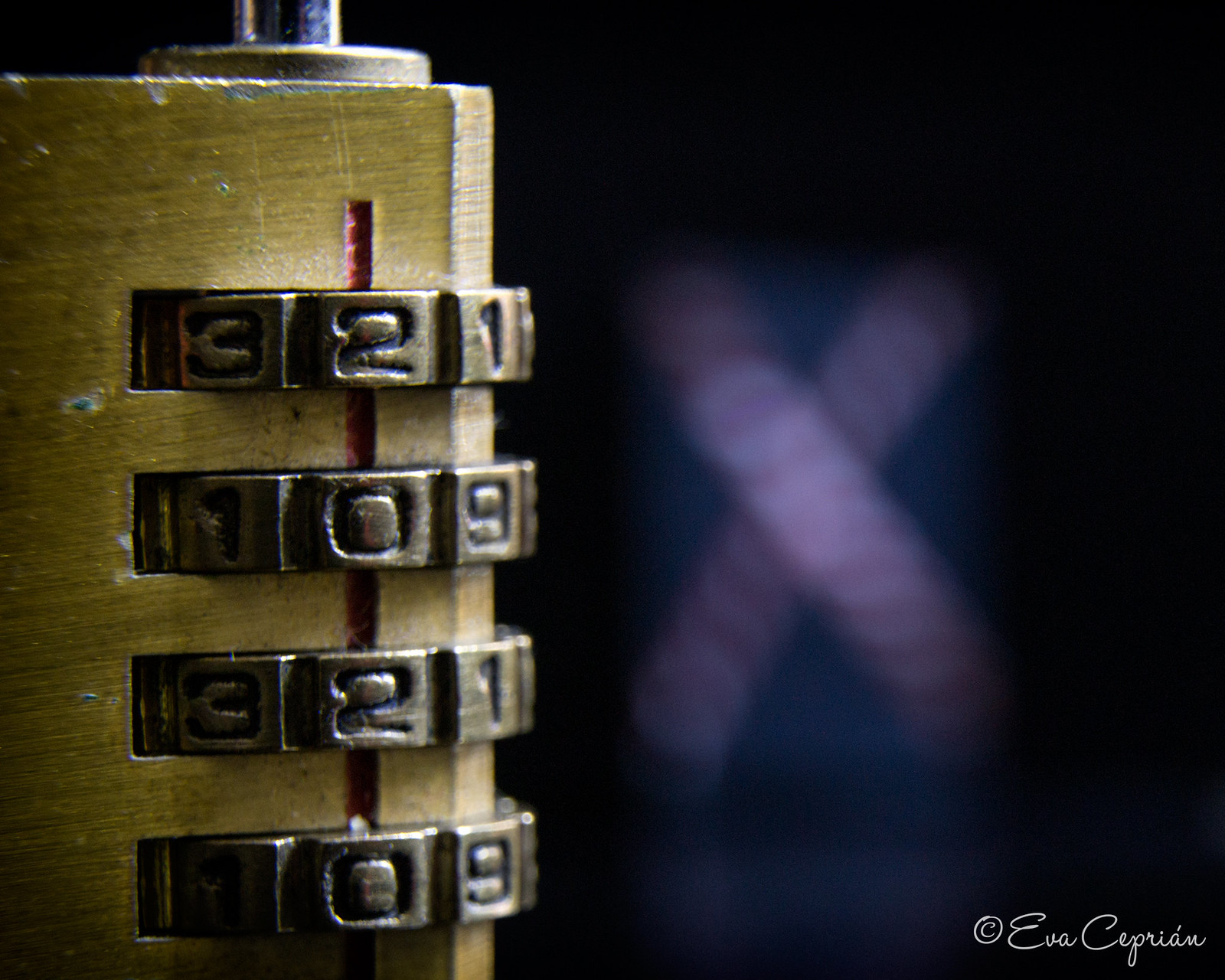This detailed image features a silver gunmetal-colored combination lock with a slightly chipped surface, revealing darker patches. The lock is affixed to a piece of brown wood and has distinctive red strips marking the number dials. The code sequence on the lock reads 3-2-1, 1-0-9, 3-2-1, 1-0-9, repeated across the four number slots. In the background, there is a blue wall adorned with a prominent, candy-cane-striped red and white X shape. Also, a rectangle with black and reddish silver intersecting lines forms an X pattern on the right-hand side. The bottom right corner of the image holds a copyright symbol (C), followed by the name "Eva Céprian" in script, indicating the photographer.